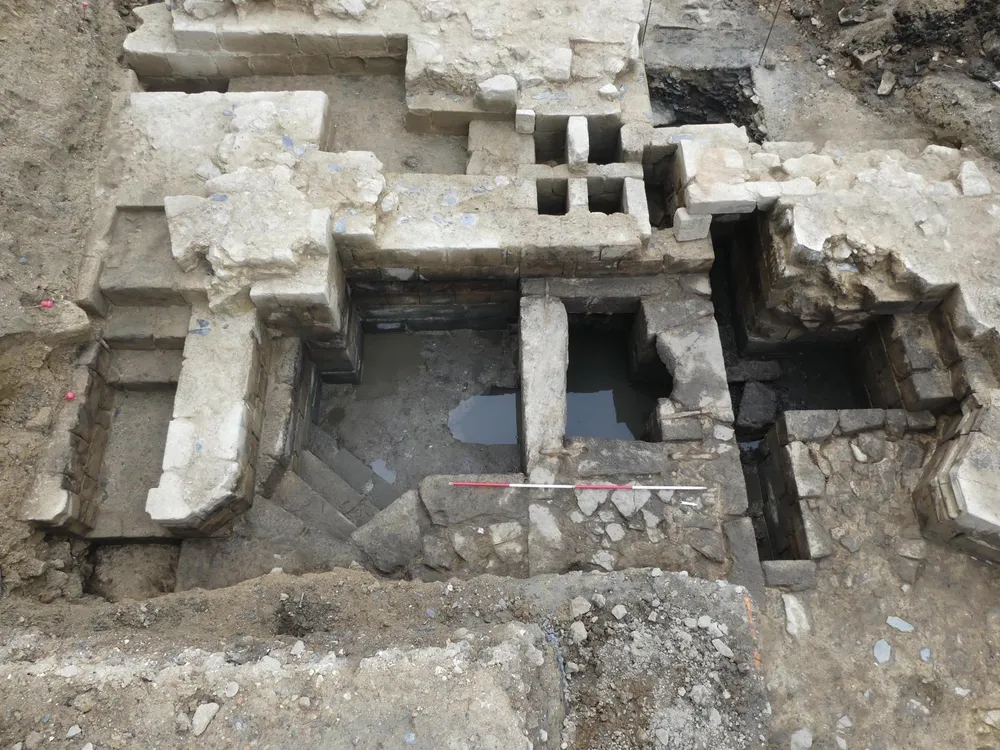The image depicts a top-down view of an excavated archaeological site resembling ancient stone ruins, possibly of a pyramid or a buried city. The scene is dominated by gray and tan stones, with black and brown mud noticeable at the bottom and the top right corner. Central to the image is a coffin-shaped pool of water, reflecting the sky above. Adjacent to this pool, at the southern edge, lies a red and white striped stick. Surrounding the water are various rock-constructed elements: staircases, walkways, and multiple window-like holes that penetrate the stone walls. The site appears to be recently uncovered and shows signs of ancient construction, possibly without a roof. Additional red objects are visible on the left side, adding a splash of color to the predominantly stony and earthen hues.